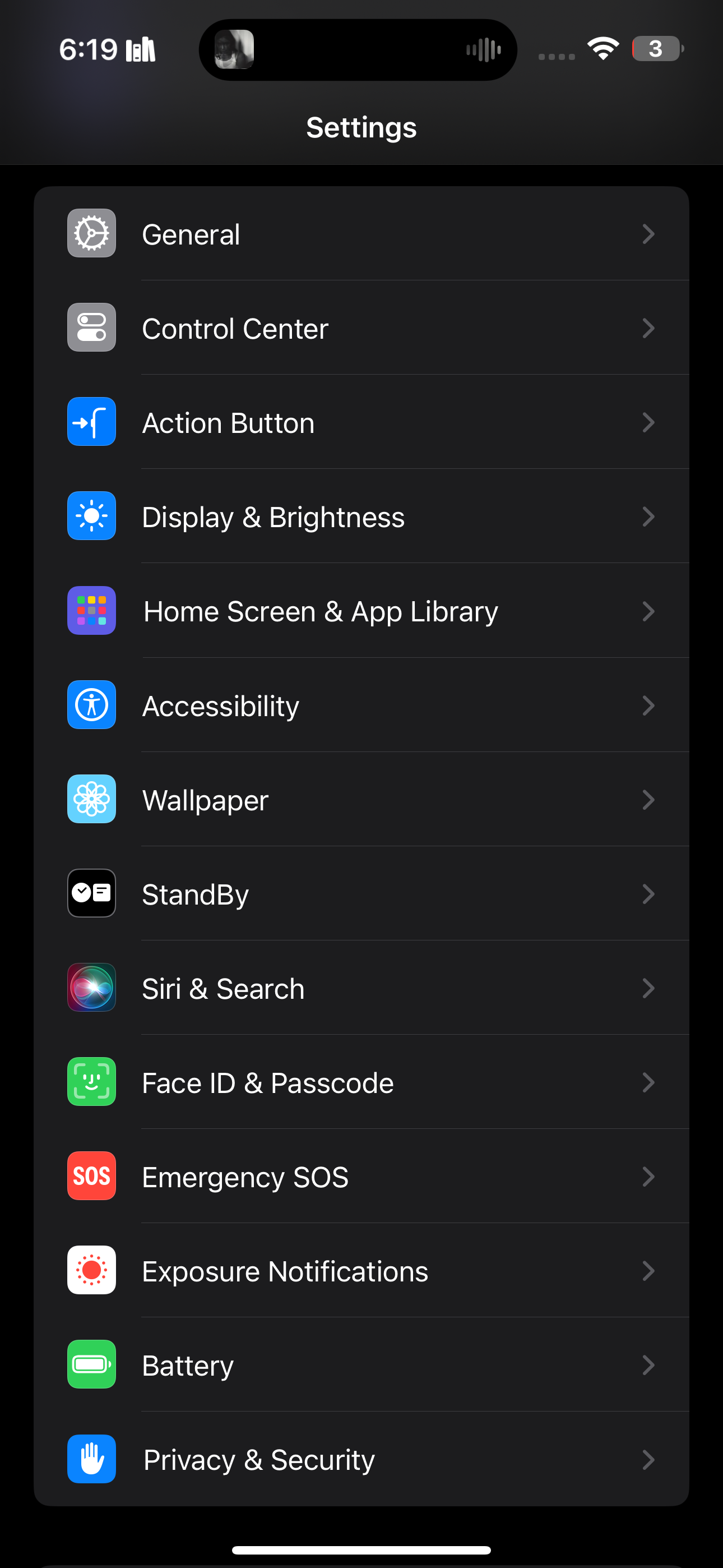The image showcases a screenshot of an iPhone's settings page in dark mode. The list prominently displays various subcategories such as General, Control Center, Action Button, Display & Brightness, Home Screen & App Library, Accessibility, Wallpaper, Standby, Siri & Search, Face ID & Passcode, Emergency SOS, Exposure Notifications, Battery, Privacy & Security. Each category is clearly labeled, offering a comprehensive overview of the available settings options. The device is shown to have only 3% battery remaining, indicated by a red battery icon in the top-right corner, alongside the time, which is 6:19, and the Wi-Fi status icon, signifying an active Wi-Fi connection. The dark mode setting provides a sleek, black background for the interface, enhancing readability and reducing eye strain.